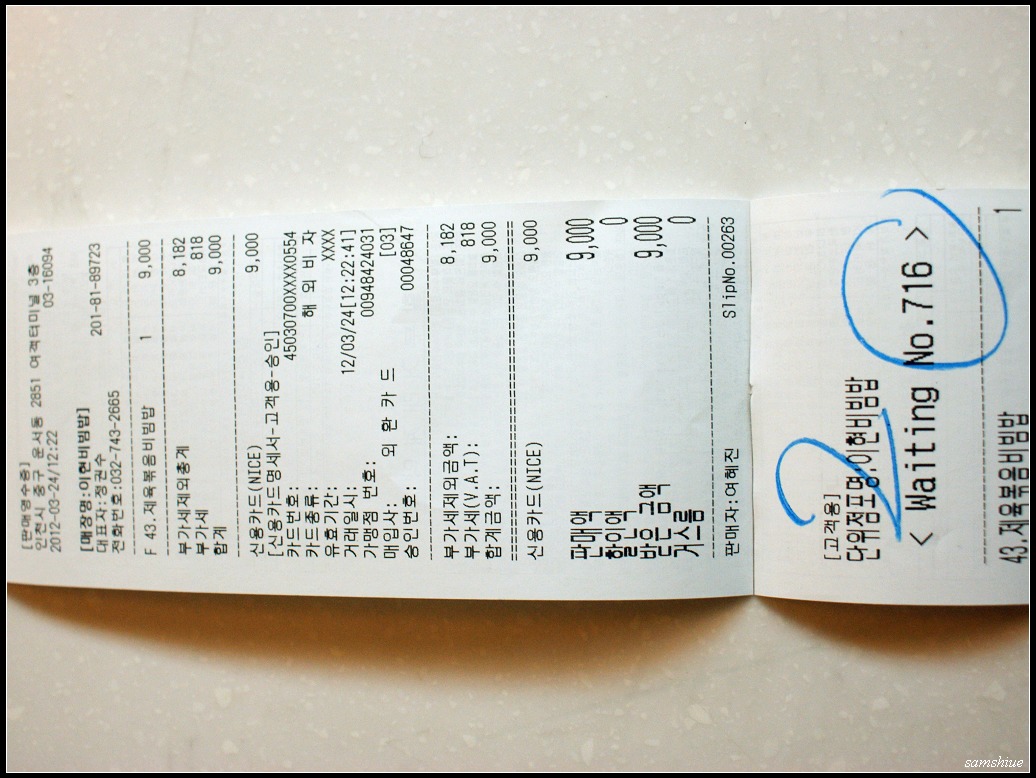This image features a horizontally oriented white receipt with primarily black text, presenting detailed information in what appear to be either Korean or Chinese characters. The date "2012 03 24" is clearly printed on the top, and the time "12:2022" is also visible. The contents of the receipt are divided by lines separating various listed items or transactions, summing up to an amount that seems to be 9,000, possibly in the local currency, like yen.

Distinctively, at the bottom of the receipt, there is the phrase "Waiting number 716," which is underlined using blue marker with the number "20" handwritten alongside it. The receipt shows signs of handling, including a noticeable fold about a quarter way up the paper. The background in the image includes a beige-colored countertop that provides contrast to the stark white of the receipt, enhancing the visibility of the text and markings. Overall, this image documents a receipt with significant annotations and a thoughtful organizational layout.